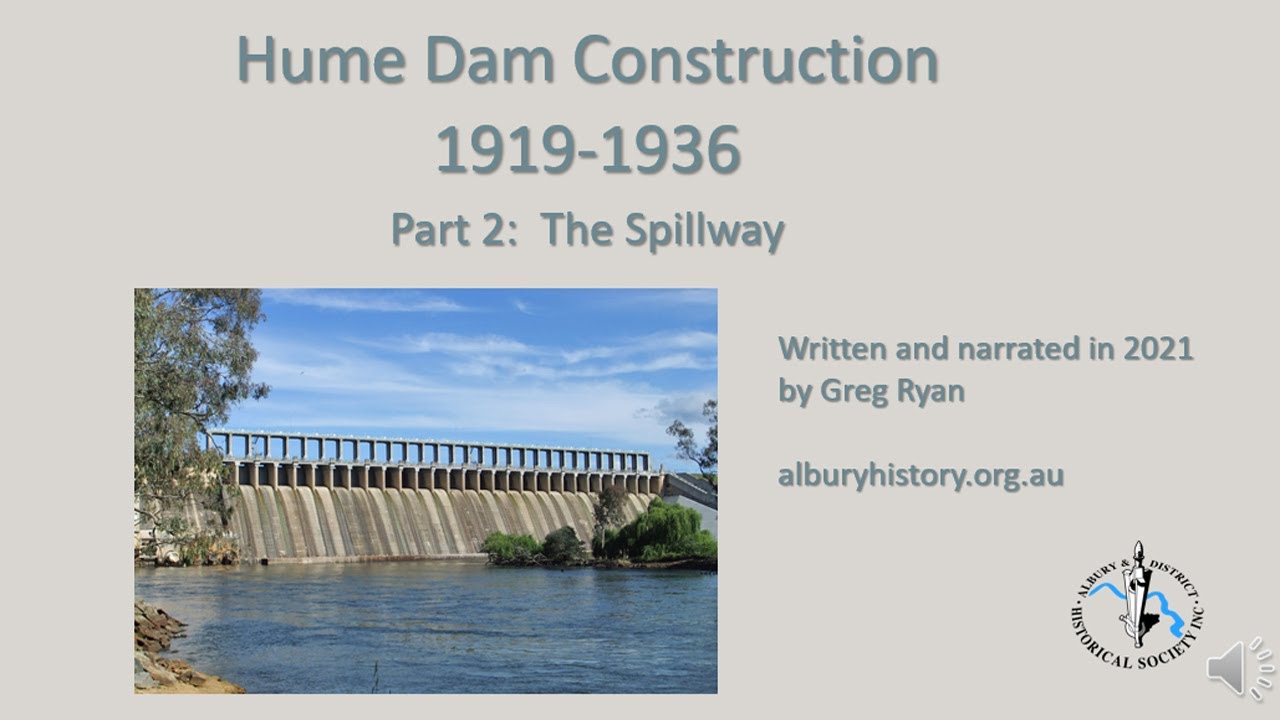The image is an interactive presentation about the Hume Dam Construction, spanning the years 1919-1936. The background is light gray with grayish-teal text. At the top center, the text reads "Hume Dam Construction 1919-1936 Part 2 The Spillway." Written and narrated in 2021 by Greg Ryan, the presentation is associated with alburyhistory.org.au. The centerpiece of the graphic is a picture of the Hume Dam located in the bottom left. The dam stretches across the image, with calm water in front and trees lining the banks. The sky above the dam is blue with white clouds. On the right side of the image, there's text stating "Written and narrated in 2021 by Greg Ryan." The website alburyhistory.org.au is also mentioned nearby. A logo for the Albury District Historical Society, Inc. appears in the bottom right corner, accompanied by a small speaker icon.